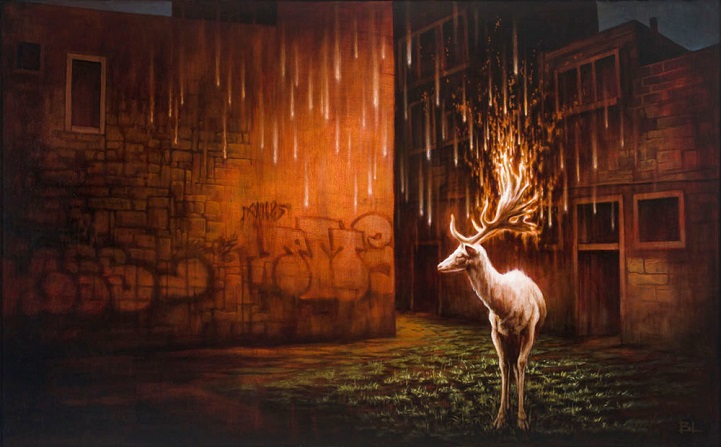The image portrays a fantastical scene set at night, featuring a majestic white deer (or stag) with golden-yellow, flaming antlers that illuminate the surroundings. The deer is positioned slightly to the right and lower part of the image, standing on a small patch of green grass. The scene appears to be in an alleyway flanked by old, worn-down buildings. To the right of the deer, you can see these deteriorating structures, some of which are partially in the shadows, creating gray and black tones. On the left side of the image, a building extends all the way up to the top left corner, featuring some visible graffiti. Raindrops are visible, adding to the night-time atmosphere. The overall setting and style of the image suggest a digitally created, fantasy environment.